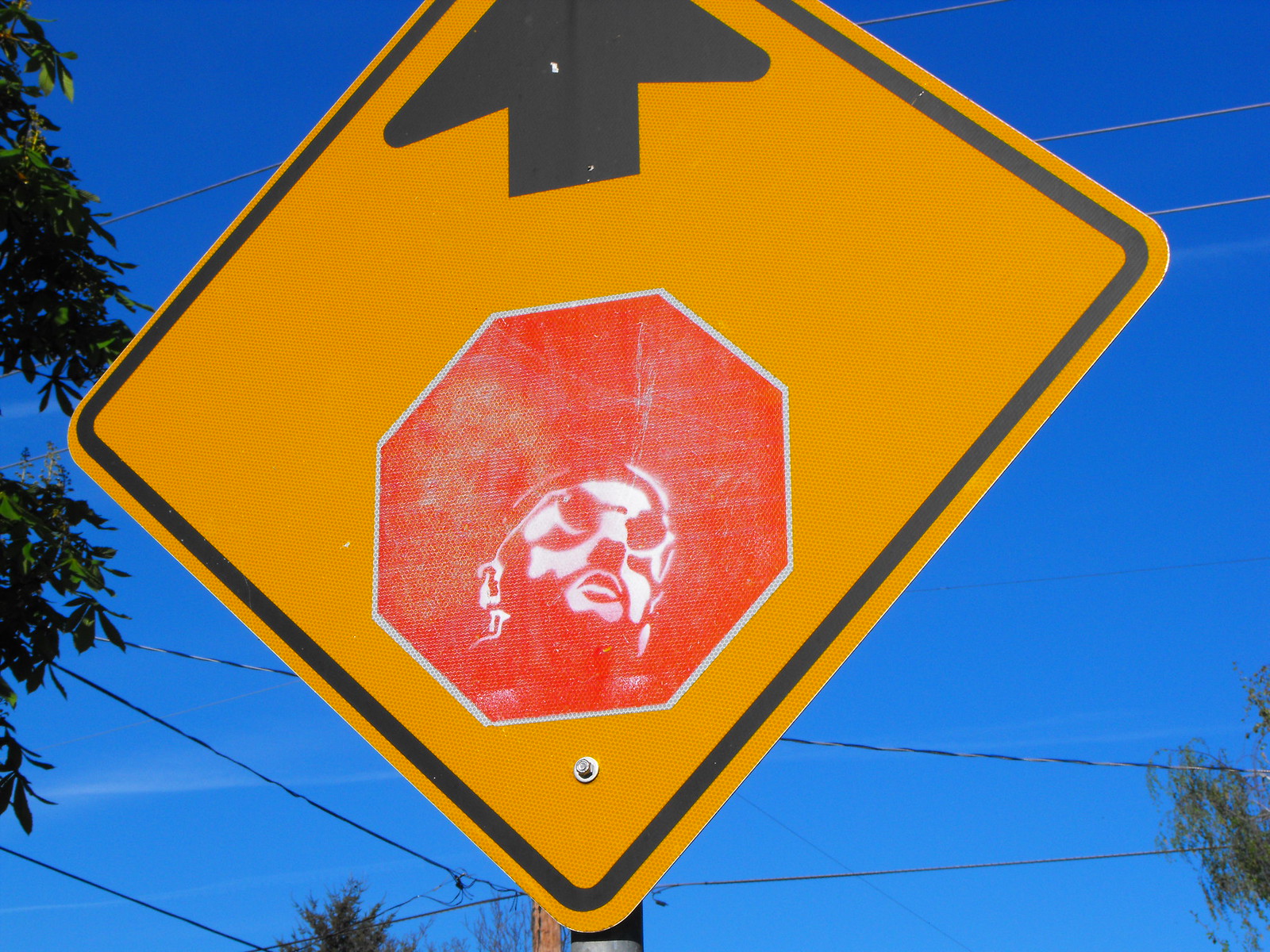A vibrant urban street scene featuring a diamond-shaped yellow traffic sign with a black border prominently displayed. The sign is adorned with a black arrow pointing upwards, symbolizing the direction of travel. Centrally affixed over the arrow is a distinctive red stop sign, adding a striking contrast. Intriguingly, the stop sign features graffiti-like artwork depicting a man's face, with notable facial highlights including his lips and the whites of his ears and face. Darkened areas suggest facial hair, giving the artwork a vivid, gritty texture. The backdrop showcases a bright, almost surreal blue sky. Electrical lines run horizontally behind the sign, adding an element of urban realism. Surrounding the sign are lush, green trees that contrast nicely with the blue sky and the vibrant colors of the sign, creating a visually captivating composition filled with dynamic hues of green, blue, yellow, and red.